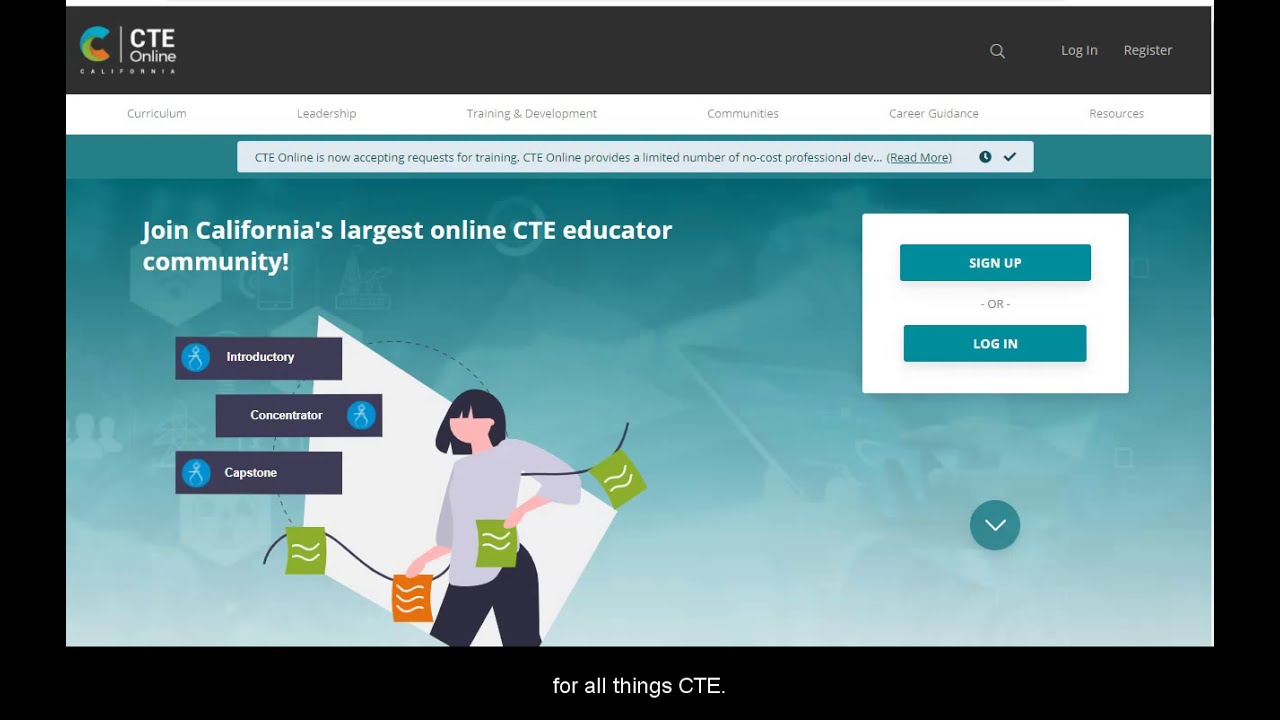A cropped screenshot of a website, depicting the interface of CTE Online. In the top-left corner, "CTE Online" is prominently displayed alongside a logo. Adjacent to this, aligned to the right, sits a search bar followed by small white-font links for "Login" and "Register." 

Directly beneath, a white bar stretches horizontally across the screen, listing categories such as Curriculum, Leadership, Training and Development, Communities, Career Guidance, and Resources. A pop-up below this bar announces that "CTE Online is now accepting requests for training," accompanied by additional information and a check mark on the right.

The main body of the page features a blue background adorned with white silhouetted images. On the bottom left, clipart depicts a woman holding a banner. Next to her are three black boxes labeled Inventory, Concentrator, and Caption.

In the top-right section, a small white box contains blue buttons labeled "Sign Up or Log In," with a downward arrow suggesting a drop-down menu beneath it. Enclosing the left, right, and bottom borders of the page is a thick black banner. Centered at the bottom of this black border, an edited text reads, "For All Things CTE."